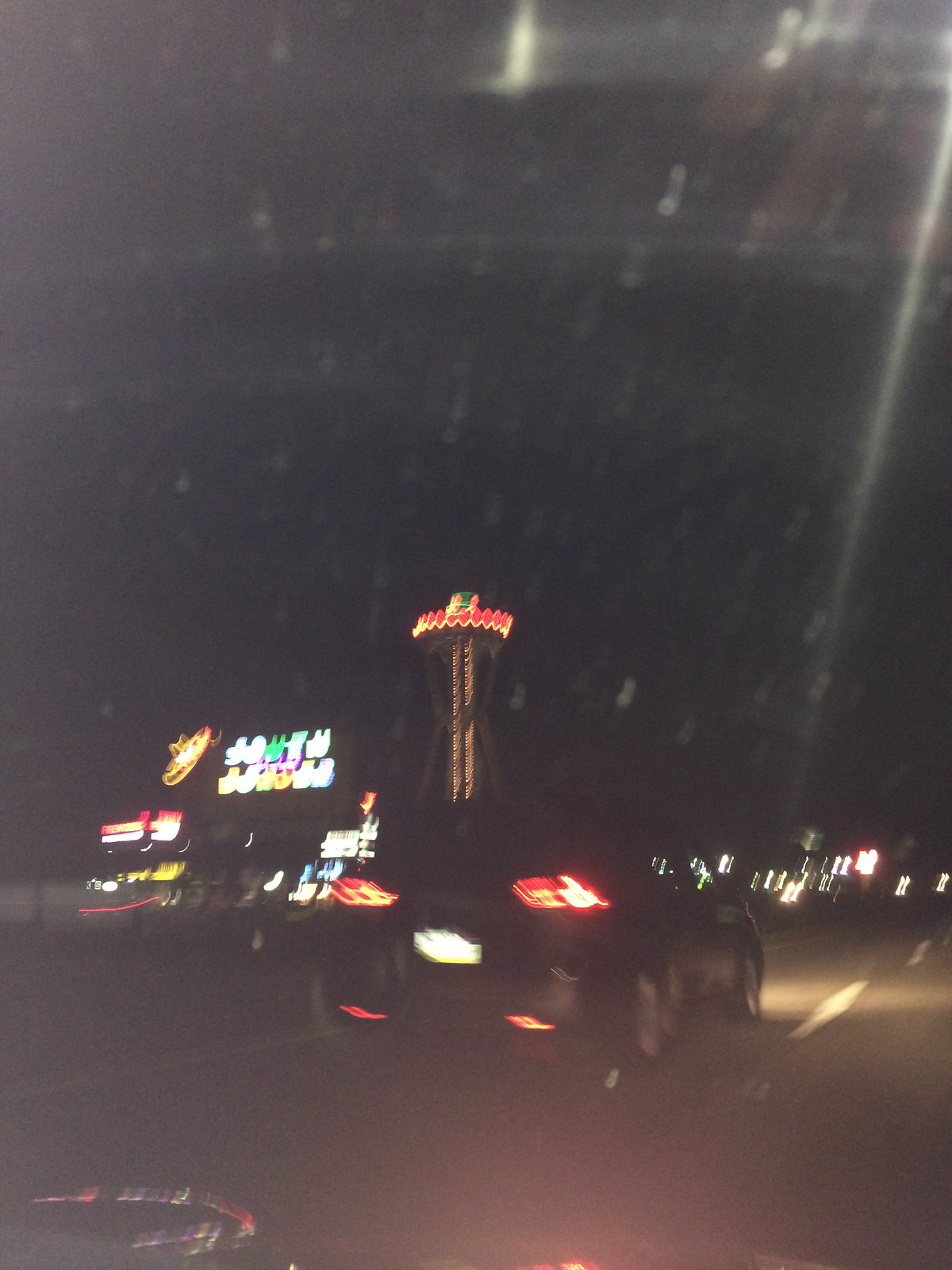This blurry, nighttime photo captures a scene from a moving vehicle on a highway, likely taken through a windshield or driver's side window. In the foreground, a black car with its brake lights on is visible in the left lane of a two-lane road, delineated by a white dotted line. The car’s rear lights and a blurry license plate are discernible, along with additional lights underneath the plate. The image is marked by poor quality and light reflections across the lower part of the frame and possibly due to dirty glass.

On the horizon to the left, illuminated city structures suggest we might be in a place like Las Vegas or Reno. There's a brightly lit, tall tower featuring red and yellow lights toward its top, and a sign resembling a sombrero with neon writing, indicating a casino or similar establishment. Bright lights and the general cityscape, including additional lighted structures, add to the urban nighttime atmosphere.